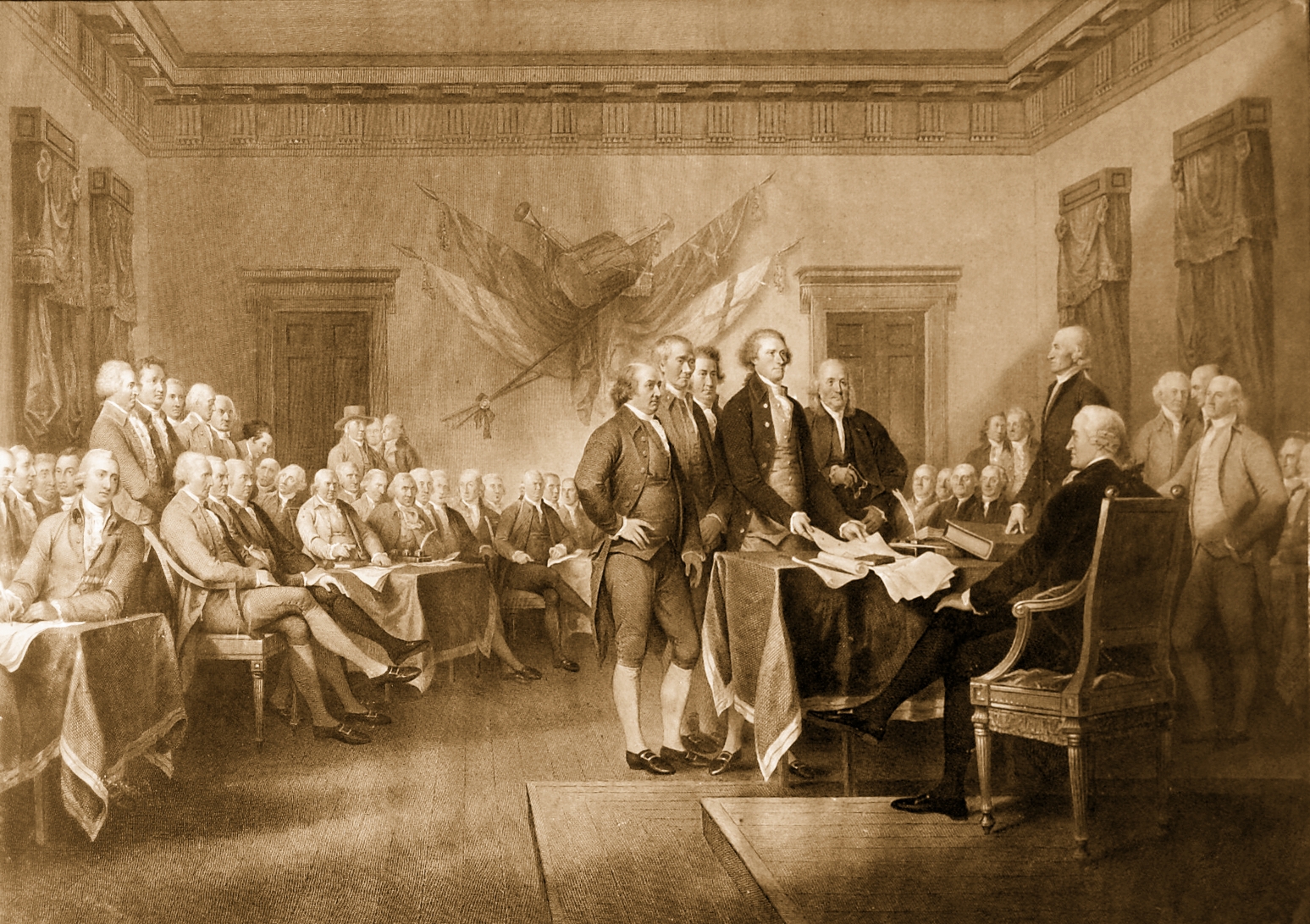This artistic piece appears to be a detailed sketch or painting, rendered in a brown, goldish tint, possibly depicting a scene from the 17th or 18th century, akin to the signing of the Declaration of Independence. The setting is an interior room with a white far wall adorned with multiple crossing flags and flanked by large square rectangular windows with closed curtains. The side walls are also white, each featuring two tall windows.

Central to the scene, a man dressed in black sits behind a desk draped with a dark tablecloth edged in white. His white hair suggests he might be a person of importance. The desk is cluttered with several documents, a feather quill, an inkwell, and a book. In front of the desk, five men stand, holding documents, with attire characteristic of the George Washington era, including white wigs, collared shirts, high white socks, and varied coats in shades of brown and darker hues. One man stands with his arm on his hip, while another barely visible figure suggests more individuals involved in this historic gathering. The floor indicates a basic square stone design, and two doors are present on the back left and right sides of the room. The men on the left side, seated with legs crossed, share similar white wig styles, light brown suits, and tights, while those on the right side, both standing and seated, mirror this attire, contributing to the solemn atmosphere of this pivotal meeting.